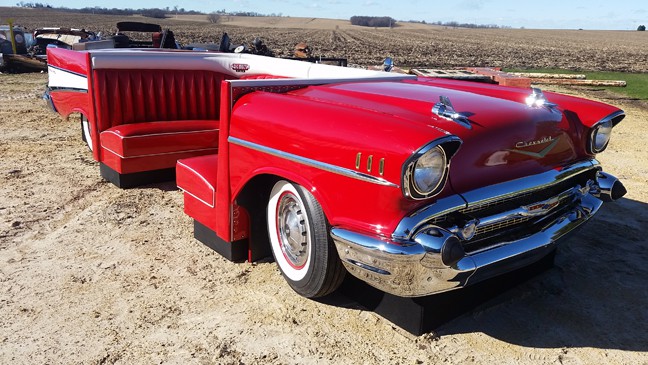This is an outdoor daytime photograph capturing a meticulously transformed vintage red convertible, possibly from the 1950s or 60s, that appears to be a Chevrolet or Cadillac. The classic car features distinctive chrome bumpers and black tires with white walls. Its roof and windshield have been removed, and the interior has been artfully converted into a diner-like booth with red leather seats arranged face-to-face, suggestive of a cozy dining area. The car's exterior includes a silver front fender with a white stripe adorning the back, adding to its retro charm. The setting is a dirt-packed field, with freshly tilled earth visible in the background. To the right, wooden logs lay scattered on the grass, and assorted machinery and deconstructed vehicles pepper the landscape, hinting at the scene being an old automobile junkyard. The photograph, roughly four inches wide by three inches high, captures a nostalgic yet inventive repurposing of automotive history.